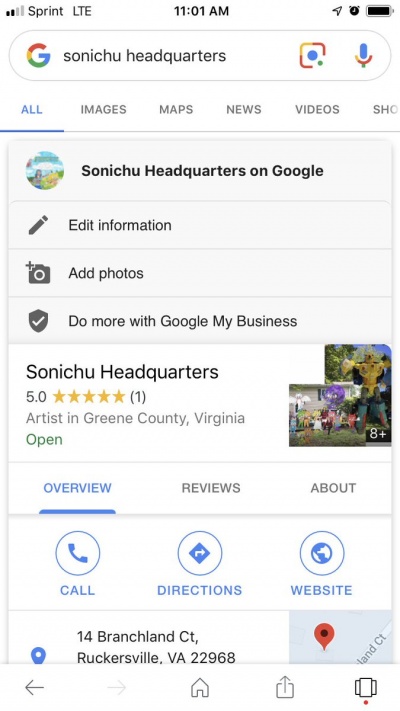This is a detailed screenshot from a tablet or cell phone displaying a Google search. The device shows a signal strength of 2 out of 4 bars with LTE connectivity, and the current time is 11:01 AM. The battery is fully charged, and an alarm is set. 

On the screen, the Google search bar contains the query "Sonichu headquarters". The 'All' tab is selected and highlighted in blue, with other tabs available including Images, Maps, News, Videos, and another partially visible option starting with "SHO".

Below the search bar, the screen displays information about "Sonichu headquarters." Options are available to edit information, add photos, and utilize Google My Business features. The headquarters are rated 5 stars based on a single review, labeled as "Artist in Green County, Virginia" and currently open. Although 8 photos are available, they are not visible in the screenshot.

The overview section is highlighted, providing the address: 14 Blanchard CT, Rockersville, VA 22968. There is also a link to Google Maps for navigation to the location.